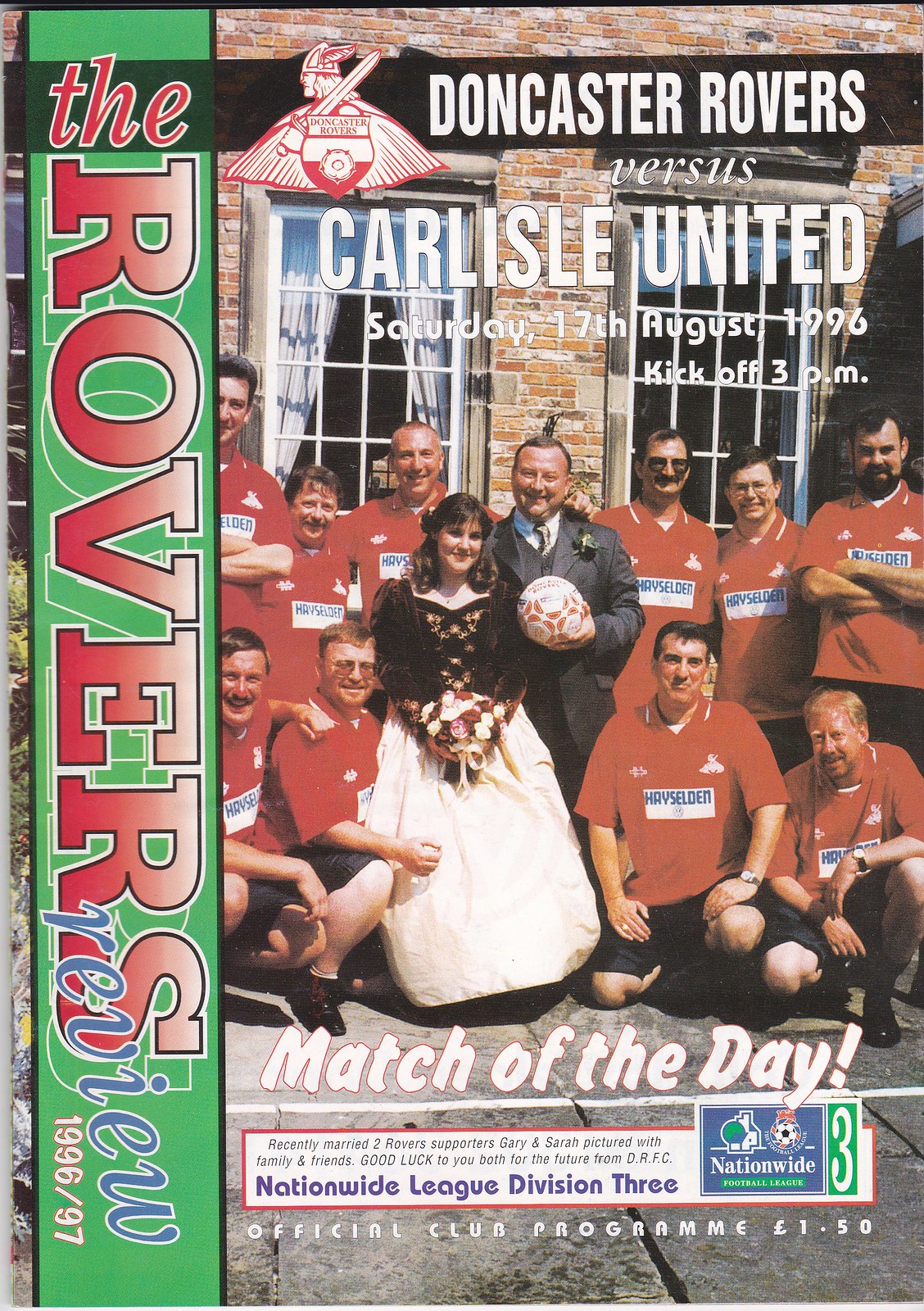The tall rectangular image showcases the front side of a sports magazine, with a background featuring an older group of soccer players wearing red jerseys adorned with a logo. In the center, a woman dressed in a long white skirt and a brown velvet shirt with gold patterns holds a bouquet and stands slightly in front of a larger man in a gray tuxedo, who is holding a white and red soccer ball. This duo is flanked by four seated individuals and additional standing players. To the left of the page, a tall green rectangle runs vertically, reading "ROVERS REVIEW" in red gradient, all capital letters. The top headline announces "Doncaster Rovers versus Carlisle United, Saturday, 17th of August, 1996, kickoff at 3 p.m." Below the photo, text declares "match of the day" and indicates this is the "official club program" for the National League Division III. The image also includes partially visible elements such as a brick building with two windows in the background.